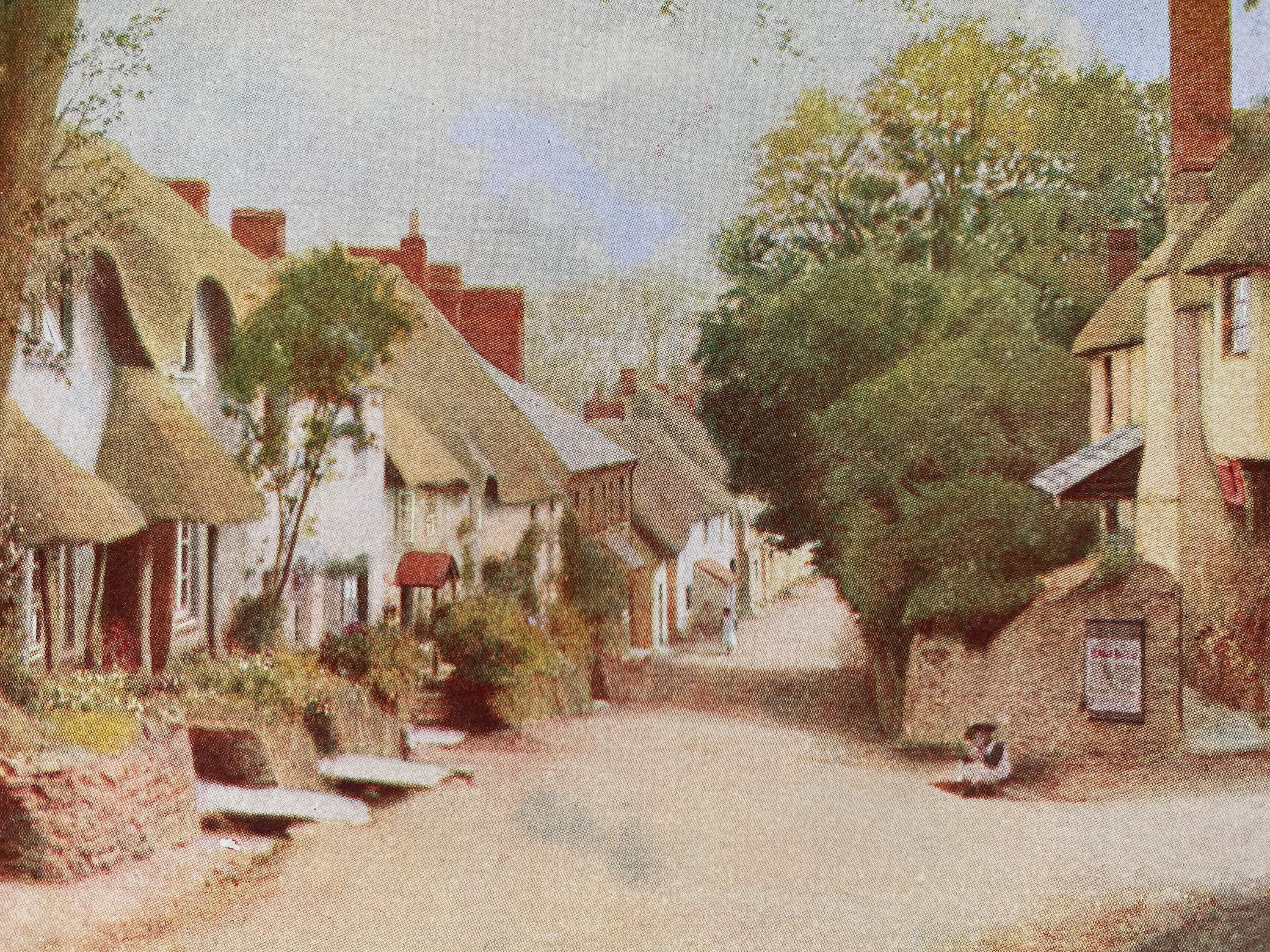The image depicts an old, quaint village, possibly from the 1800s, with a European ambiance, perhaps Dutch. The painting is rendered in a style reminiscent of pointillism with fuzzy and grainy textures, using very light brush strokes that give it an antique feel. The scene features a long, stone or brick boulevard gently sloping downhill, flanked by houses and trees. The buildings are varied in color—white, tan, and brick—with moss or grass-covered roofs, some topped with red chimneys. 

Green foliage and flowers are prevalent, adding vibrant accents against the numerous brick-fronted homes and apartments. Among the notable features are awnings and white walkways leading to the houses, with high porches and small yards where white flowers grow. There is a pathway lined with a brick wall that leads up to the porches, reinforcing the village’s charming character.

Two small figures are present in the scene: to the right, a person dressed in a hat is sitting on the ground underneath a sign, and further down the boulevard, near a shadowy area, stands another figure, possibly a female. The sky above is cloudy, adding a serene atmosphere to this picturesque village landscape.